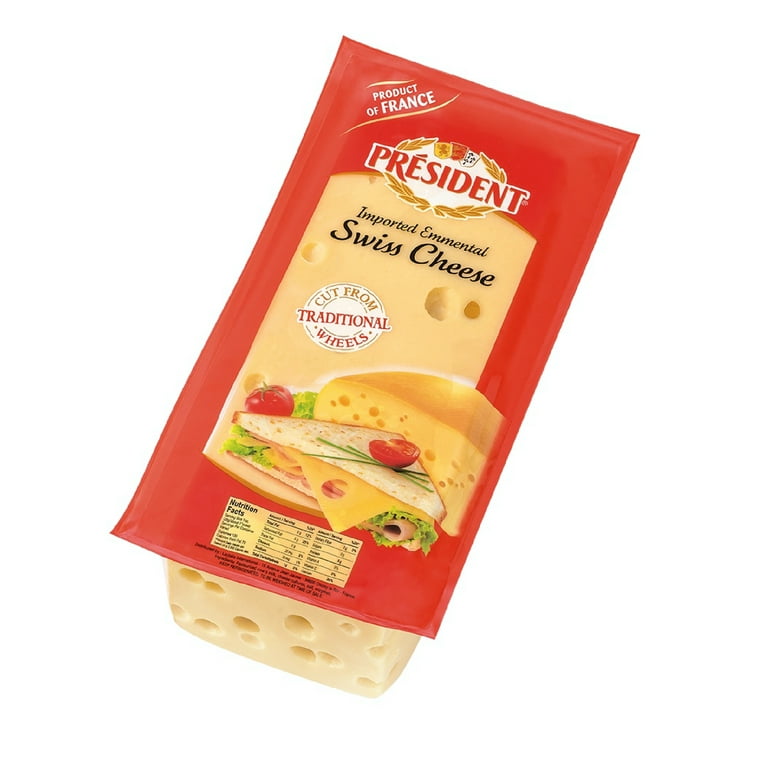The photograph shows a package of Swiss cheese, specifically President brand imported Emmental Swiss cheese cut from traditional wheels, with text noting it is a Product of France. The cheese package features a primarily red label that includes an oval-shaped logo with "President" inside a laurel wreath. The label presents a detailed image of a cheese wheel cut in half, revealing its holey texture, with a half sandwich placed diagonally in front of the wheel. The sandwich, garnished with a tomato slice, green leafy strips, ham, lettuce, and Swiss cheese, is accompanied by a whole tomato and some lettuce on the left side. The bottom portion of the package is transparent, allowing a clear view of the white Swiss cheese block with its characteristic holes. Nutritional facts are printed in very small font at the bottom of the packaging. The transparent window at the top of the packaging further reveals the texture and dimensions of the cheese.